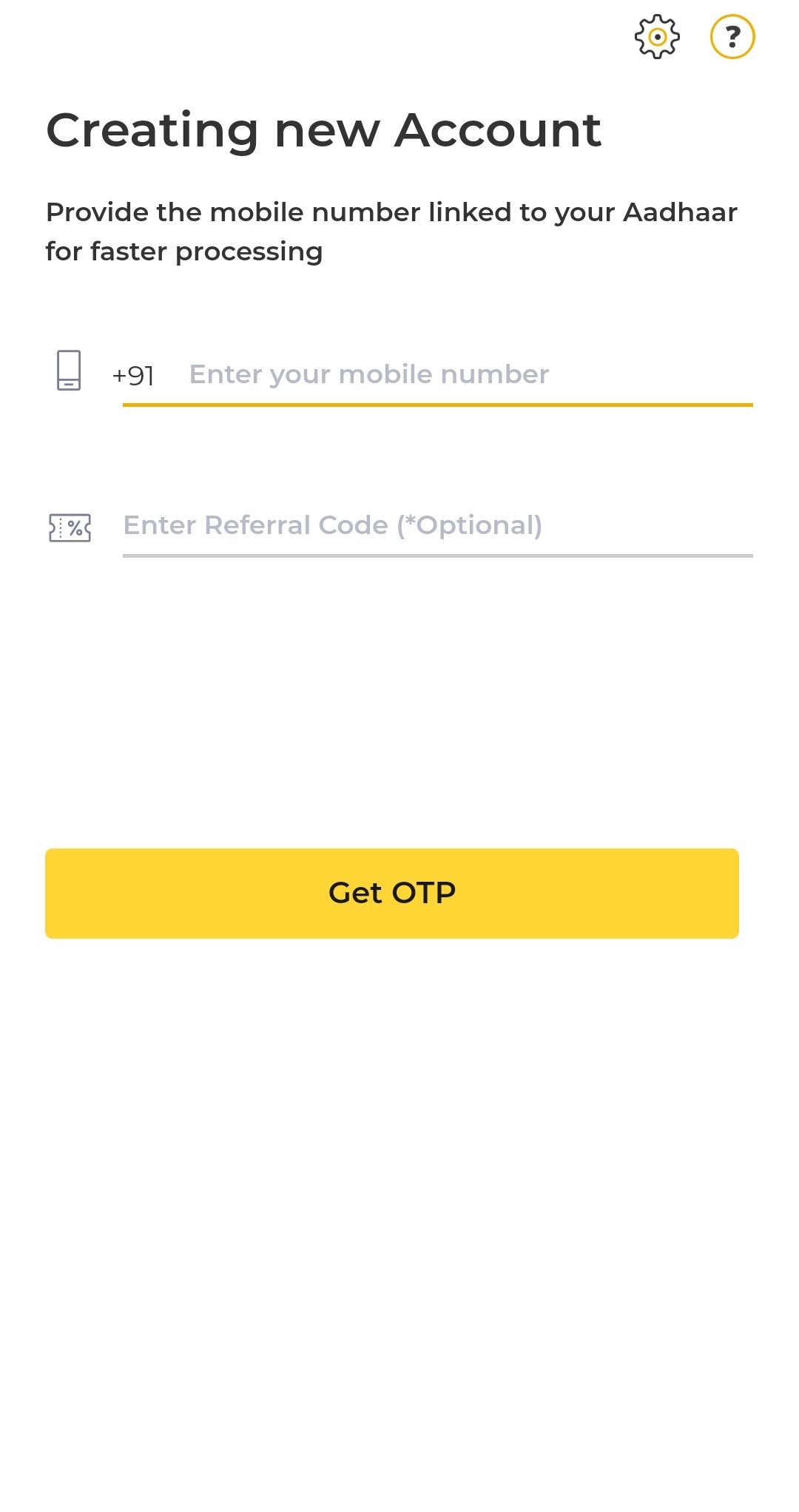The image presents a minimalistic interface on a white background, primarily focusing on account creation. At the top, the text "Creating New Account" is displayed in black. Below it, a prompt reads: "Provide the mobile number linked to your Aadhaar for faster processing," with "Aadhaar" specifically spelled with an uppercase "A" and lowercase "aadhaar."

An outlined cell phone icon is situated beneath the prompt, which displays the country code "+91." Adjacent to this icon, there's a light gray placeholder text saying "Enter your mobile number," underlined with a yellow line, indicating that user input is awaited.

Further down, a subtle light gray text and accompanying ticket symbol provide a field for "Enter Referral Code" with an asterisked note "(optional)," also underlined in light gray due to the field's inactive status.

Towards the bottom, a prominent, elongated yellow rectangle button is present with the text "Get OTP" written in black.

In the upper right corner, two icons are visible: a black gear symbol and a black question mark encased in a white circle outlined in yellow, indicating settings and help options respectively. No additional text or elements clutter the clean and straightforward design.